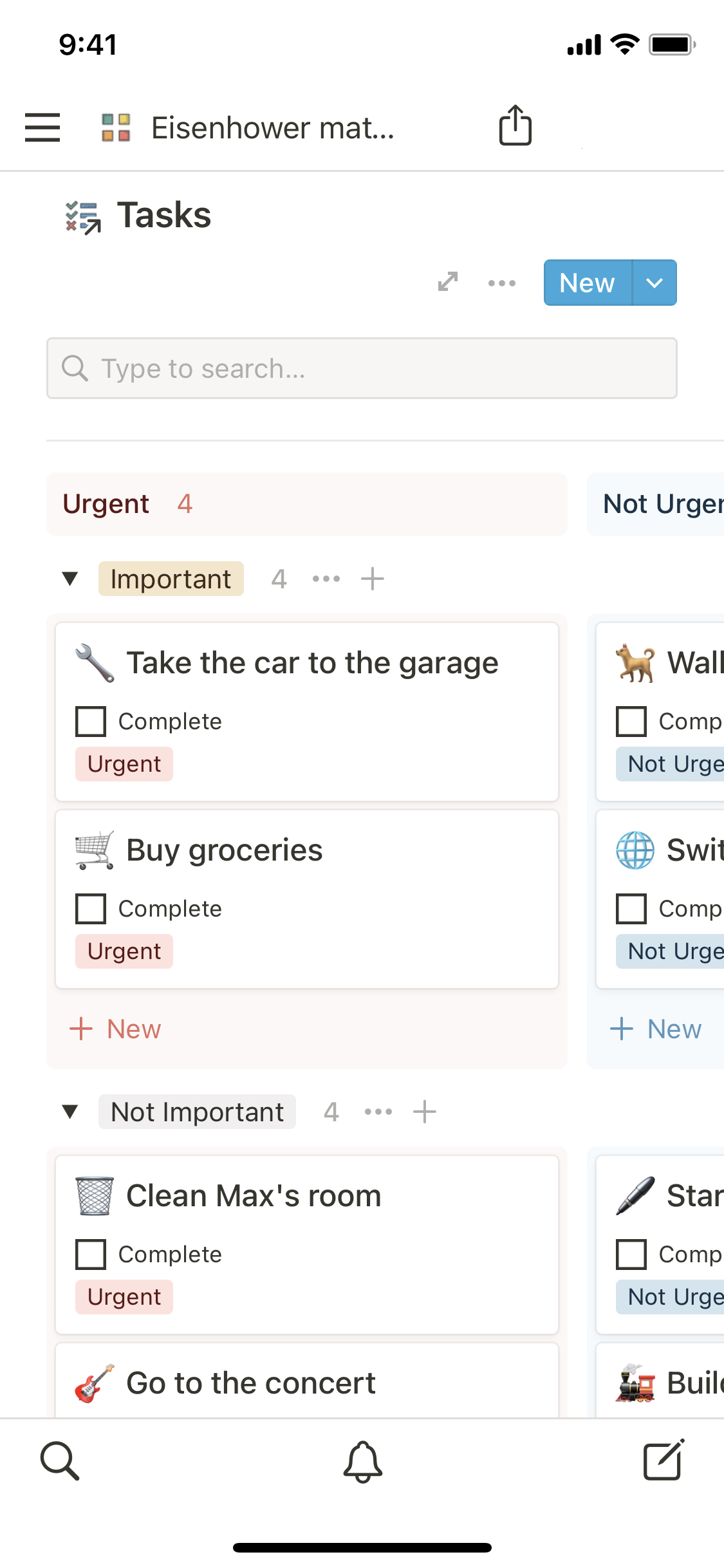Screenshot of a task management app displaying a detailed list of tasks organized by urgency and importance. The most urgent and important task is "Taking the Car to the Garage," followed by "Buying Groceries." Less critical tasks include "Cleaning Max's Room" and "Booking Concert Tickets." The app categorizes tasks into four important and four less important items, illustrating a clear prioritization strategy.